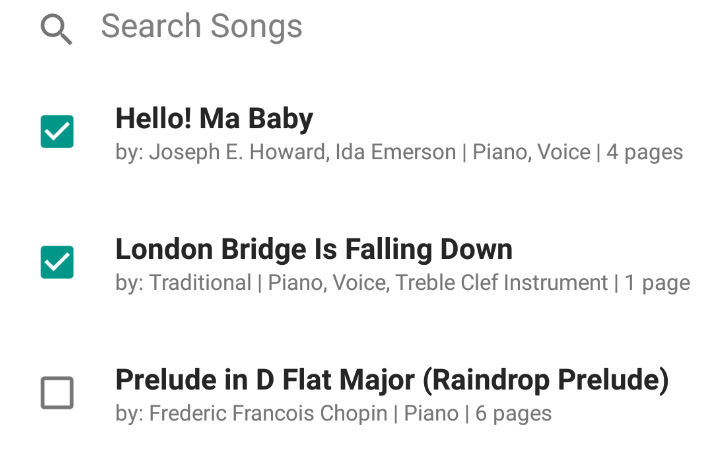This image captures a screenshot of a musical application interface on a computer. At the very top, there's a magnifying glass icon accompanied by the text "Search songs" in grey, indicating a search bar.

Below the search bar, three songs are listed in black and grey fonts. The first two songs have a white checkmark within a small green box to their left, signifying their selection. The details are as follows:

1. The first song titled "Hello Ma Baby" is presented in black text. Beneath the title, in grey text, it specifies the contributors as "by Joseph E. Howard, Ida Emerson," and mentions the format as "piano voice, four pages."
 
2. The second song listed is "London Bridge is Falling Down," also in black text. The grey text underneath indicates it is "by traditional line" with the format "piano voice, treble clef instrument, one page."

The third song, which does not have a checkmark but only an empty grey box with white at the center, is featured at the bottom:

3. Titled "Prelude in D flat major" with the subtitle "Ring Drop Prelude" in brackets, it appears in black font. The grey text below attributes the piece to "by Frédéric François Chopin" and specifies it as "piano, six pages."

The entire interface is set against a clean white background.